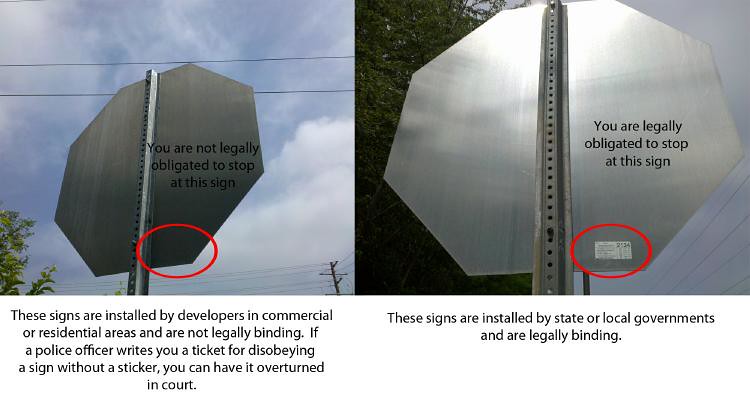The image consists of two side-by-side photographs depicting the backsides of stop signs taken on a sunny day with blue skies, clouds, numerous telephone wires, and a few trees. Both photographs illustrate the legal distinctions between certain stop signs. 

The left photograph features a metal stop sign on a pole with a red circle highlighting the absence of a sticker. Within this circle, text reads, "You are not legally obligated to stop at this sign." This stop sign is identified as one installed by developers in commercial or residential areas, which are not legally binding. The accompanying explanatory text clarifies that tickets issued for disobeying such signs can be overturned in court.

In contrast, the right photograph shows another metal stop sign on a similar pole but with a red circle around a small white rectangular sticker at the lower right. The text within the circle states, "You are legally obligated to stop at this sign." This sign type is mandated by state or local governments, making it legally binding. The explanatory text reinforces this, noting that tickets for disobeying such signs are enforceable.

Overall, these images distinguish between legally binding stop signs and those installed by developers, providing clear visual cues via the presence or absence of a white rectangular sticker.